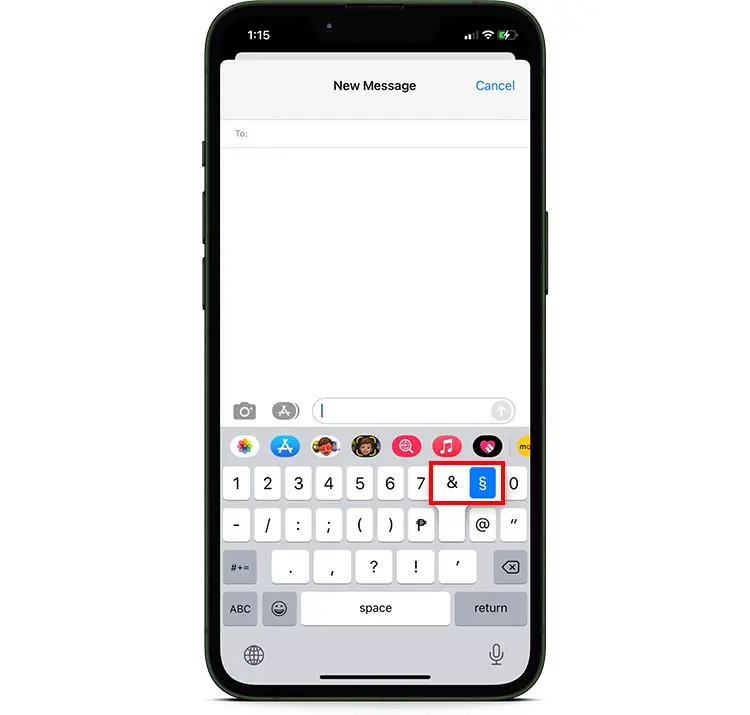The image captures a smartphone displaying a new message screen. In the top right corner, a "Cancel" option is visible. The "To" field, where the recipient's contact would be entered, is currently empty. Below it, there is a text input box, showing the on-screen keyboard.

The keyboard featured on this smartphone is quite unique and not in the usual QWERTY layout. Instead, it displays numerical and special characters, with certain keys highlighted. Specifically, a red box surrounds the ampersand ("&") and another character that resembles an ampersand but has a blue border around it, indicating their importance or a specific requirement to type them. These characters are positioned between the numbers 7 and 0 on the keyboard.

Above the keyboard, a row of app icons is displayed, including a music icon (musical notes inside a red oval), a heart symbol, a magnifying glass icon, among others. These icons appear to provide quick access to various apps or functions directly from the messaging interface. The keyboard itself presents a subset focusing on numeric and special characters, with an option labeled "ABC" for switching to alphabetic characters.